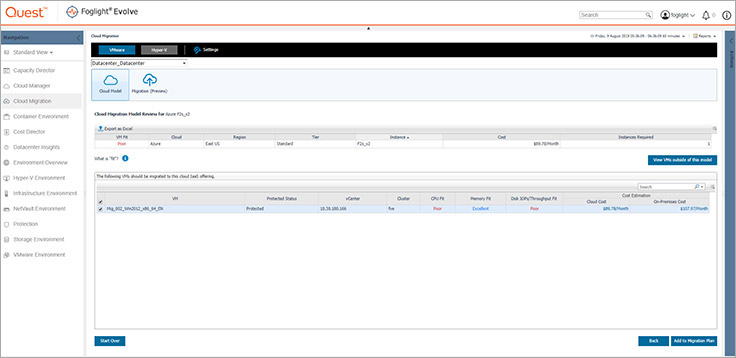The image depicts a website interface featuring a detailed layout. At the top left corner, the brand name "Quest" is displayed in prominent orange text with a capital "Q." Adjacent to it, the label "Foglight Evolve" appears in sleek black text. Moving towards the right, there is a search bar containing the placeholder text "Tag Light," followed by a notification bell icon and an icon resembling an eye inside a circle. 

Below this header, a vertical navigation menu is positioned on the left side of the screen. Despite some of the text being faint, the menu items listed include terms like "Standard View," "Capacity Director," "Cloud Manager," "Cloud Medicaid," "Migration," "Container Environment," "Cost Director," "Environment Overview," "Hyper-V Environment," "Protection," and "Storage Environment." Some menu items are too light to be clearly readable.

The main section of the website displays blurred text but visually includes a variety of cloud graphics and icons, such as a cloud with an arrow pointing out of it. Additionally, there are several charts, possibly depicting performance metrics or data analytics.

This comprehensive layout suggests that the website is likely geared towards cloud management and IT solutions, offering various tools and dashboards for monitoring and managing different environments.